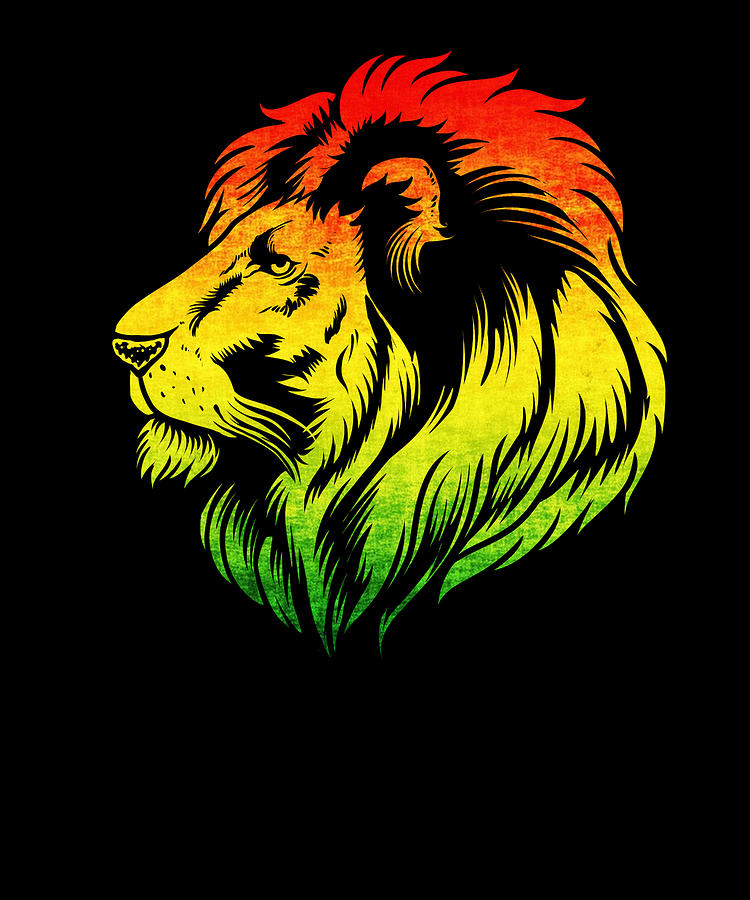The image is a detailed print or AI rendering of a male lion's head, set against a solid black background. The lion, positioned centrally and facing left, exhibits a vibrant color gradient that begins with a rich red at the top of its mane, transitions through yellow around its face, and culminates in a green hue at the bottom of its mane. The lion's ear is a striking reddish-orange, adding to the fiery palette. The intricate detailing and stylized colors, reminiscent of Jamaican themes, suggest that the artwork—whether drawn or AI-generated—could serve as a captivating logo or piece of modern digital art.